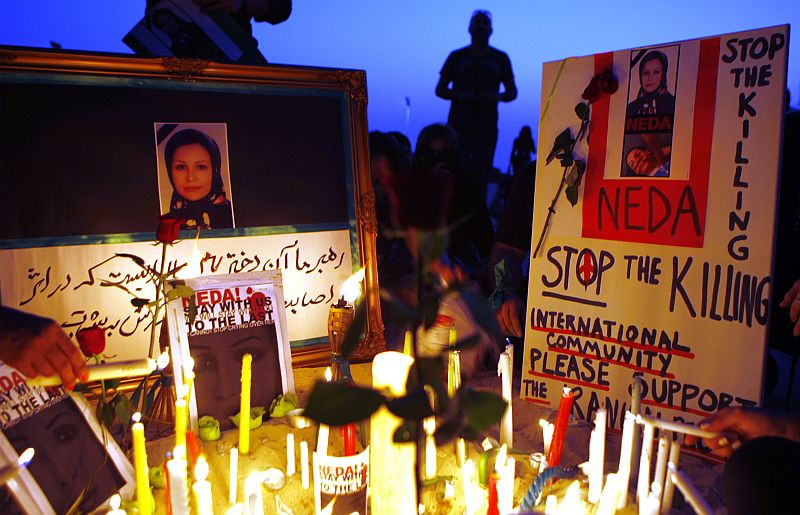The image depicts a solemn prayer vigil and makeshift memorial for a woman named Neda, showcased within a large, ornate golden wooden frame. The small photograph inside the frame shows Neda wearing a headscarf and dark attire, set against a black background. Surrounding the framed picture are numerous lit candles of various colors—yellow, white, red, and blue—situated on what seems to be a round table. To the left side of the frame is a handmade sign with a poignant plea reading in bold black letters, "NEDA, Stop the Killing" and "International Community, Please Support," partially obscured by more writing in what appears to be Arabic script. The foreground prominently features red roses with green stems, while an additional bottle labeled "Neda" is visible, hinting at a personal tribute. In the background, silhouettes of people stand and sit as dusk settles, illustrated by the blue sky transitioning to darkness. A torch, aflame with a distinct yellow light, adds to the memorial's somber atmosphere, emphasizing the collective call for justice and international support against violence in the Middle East.